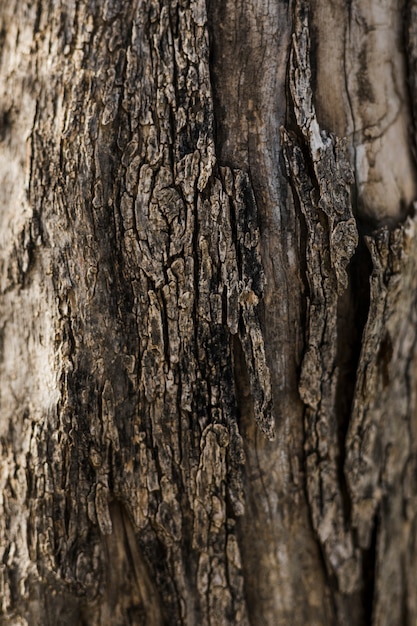This image is a close-up, detailed photograph of a tree's bark, which dominates the entire frame. The rough, craggy texture of the bark is prominently featured, with areas showing visible cracks and peeling sections. The colors range from various shades of brown to light beige, black, and gray. In the top right corner, there is noticeable bark degradation, where sections appear to be crumbling away. The overall impression is of a richly textured, natural surface, with emphasis on the tactile and visual roughness of the tree's exterior. There is no text present in the image, allowing the viewer to fully focus on the intricate details of the tree bark.